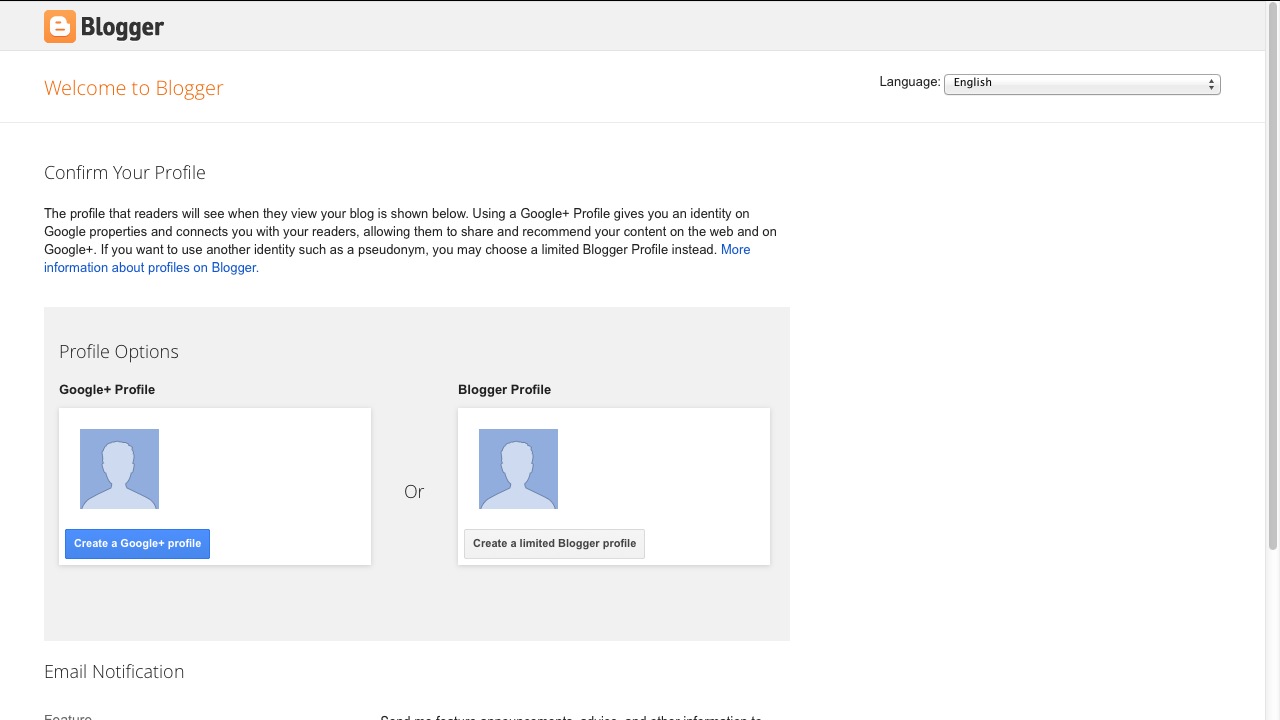The image is a screenshot of the Blogger website interface. In the top left corner, there is a small orange square featuring a white 'B', which is the Blogger icon. Right next to it, the word "Blogger" is displayed in black text. Directly below this, in bold orange text, it says "Welcome to Blogger." On the far right-hand side of the toolbar, there's a drop-down menu for selecting language preferences.

The primary focus of the screenshot is a section titled "Confirm Your Profile." Below the heading, there's a paragraph explaining that the visible profile for blog readers is shown below. It further details that using a Google Plus profile provides a recognizable identity across Google services, facilitating connections with readers and enabling them to share and recommend content via Google Plus. It also notes an alternative for those who prefer using another identity, such as a pseudonym, by opting for a limited Blogger profile instead. A link in blue text labeled "More Information About Profiles on Blogger" is provided for additional details.

Beneath this paragraph, under the heading "Profile Options," there are two profile choices: "Google Plus profile" and "Blogger profile." Both options are represented by a small blue square icon featuring the silhouette of a person. Each profile option has a clickable button to make a selection.